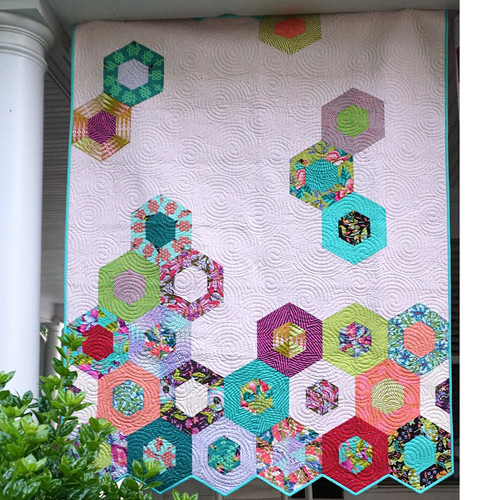In the image, a rectangular quilt hangs from what appears to be the front of a house, with a white marble pillar to its left. The quilt is bordered in aqua and has a jagged bottom edge, extending down from the roof to nearly the ground. To the lower left corner, there's a green bush or plant protruding into the frame. The quilt features an array of six-sided shapes (hexagons) that are clustered more densely at the bottom and become more dispersed towards the top, creating a sense of movement or spreading out. These hexagons are decorated in various colors and patterns, including floral designs with reds, greens, blues, yellows, peach, white, and purple, as well as specific combinations like red exteriors with blue interiors, and purple with green centers. The intricate shapes appear quilted together more tightly at the bottom, while the individual hexagons at the top leave more blank space, giving the quilt an overall dynamic and colorful appearance.